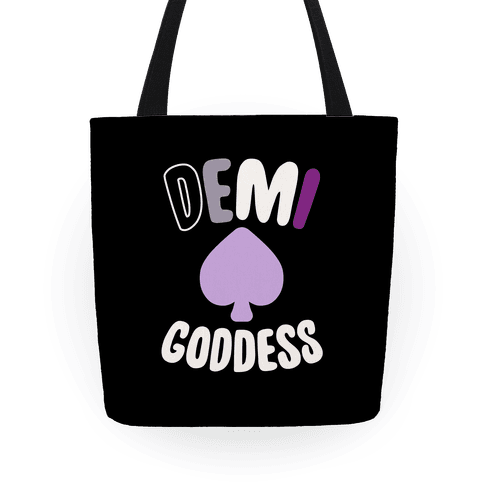A detailed illustration depicts a black tote bag with a partially visible handle extending upwards, cropped by the edge. Against a blank white background, the centerpiece of the bag is a light purple spade symbol. Above the spade, the word "Demi" is artistically rendered: the letter D is black with a white outline, the E is solid light grey, the M is solid white, and the I is dark solid purple. Below the spade, the term "Goddess" is written in uppercase block letters in solid white, arched slightly upwards. This hand-drawn artwork, which suggests it is designed for commercial purposes, highlights the bag’s potential function and aesthetic appeal.